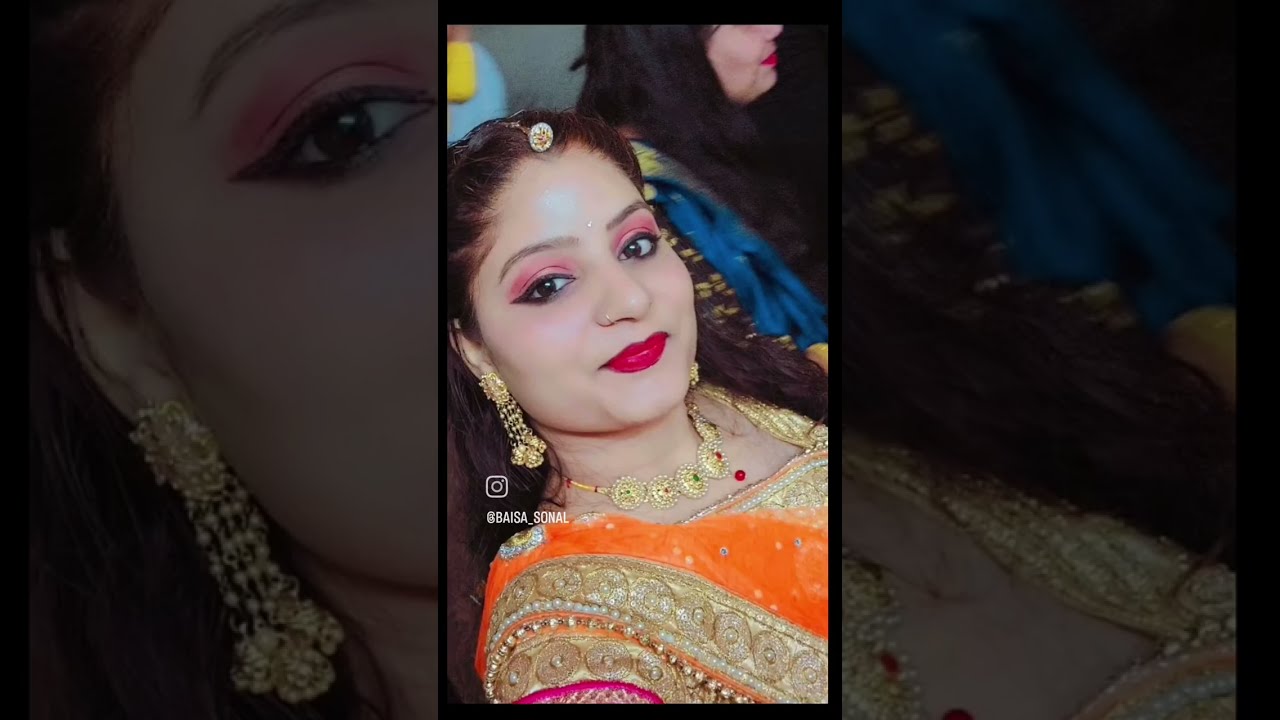This image features a close-up of a lighter-skinned Indian woman adorned in traditional attire. She is dressed formally in a sari that features a striking combination of gold, orange, and magenta stripes. Her makeup is vibrant, with pink eye shadow, heavily lined eyes, and bright red lipstick. Her round face is further highlighted by a nose ring and a charm on her forehead, connected by a chain running through the part in her black hair, which has a reddish tint and is pulled halfway back.

Her jewelry consists of gold dangly earrings and a matching gold pendant necklace made up of flat beads. She also wears other golden jewelry with hints of red and green. An orange scarf drapes around her arm, adding to the visual richness of her attire.

The background of the image is a blown-up version of her own portrait, creating a layered effect. Additionally, there is another woman in the background wearing blue with bright pink lipstick, though she is not as prominently featured. On the bottom left, there is an Instagram logo with the handle @Bicep_underscore, and the background image is darkened on the left and right sides.